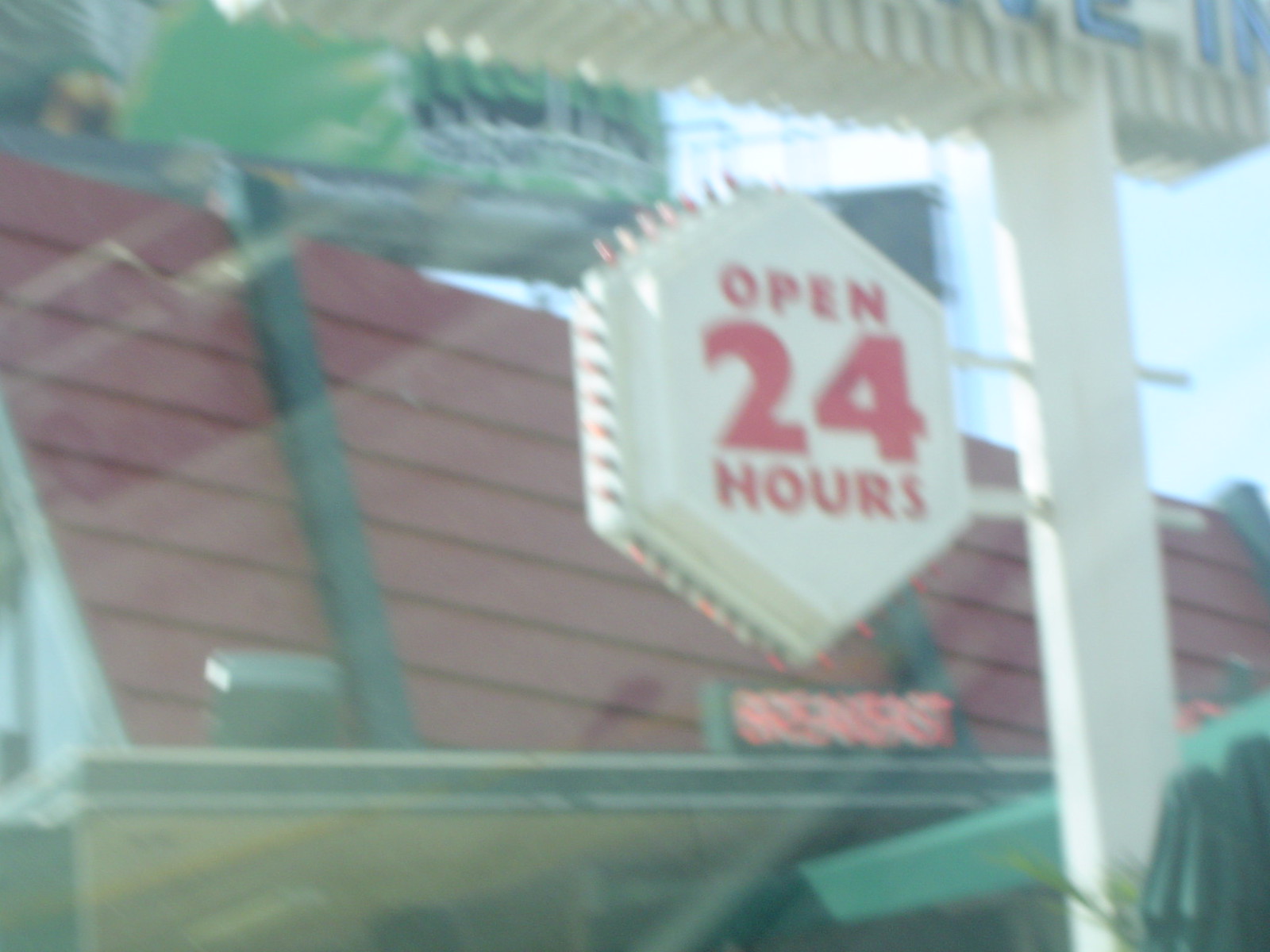A photograph captures a roadside restaurant scene through the window of a car, complete with visible reflections in the foreground. Central to the image is a uniquely shaped restaurant sign, designed to mimic a stop sign, displayed prominently on a white pole. The sign is illuminated with red bulbs lining its edges and features bold red lettering that announces, "OPEN 24 HOURS," in the center. Above this sign, the bottom edge of a larger sign peeks into the frame. The background reveals the restaurant itself, showcasing its distinctive red roof and a neon sign that reads "BREAKFAST" in glowing red letters, positioned just beneath the "OPEN 24 HOURS" sign. Black lights adorn the edge of the restaurant's roof, adding a subtle but defining touch to the overall ambiance of the scene.